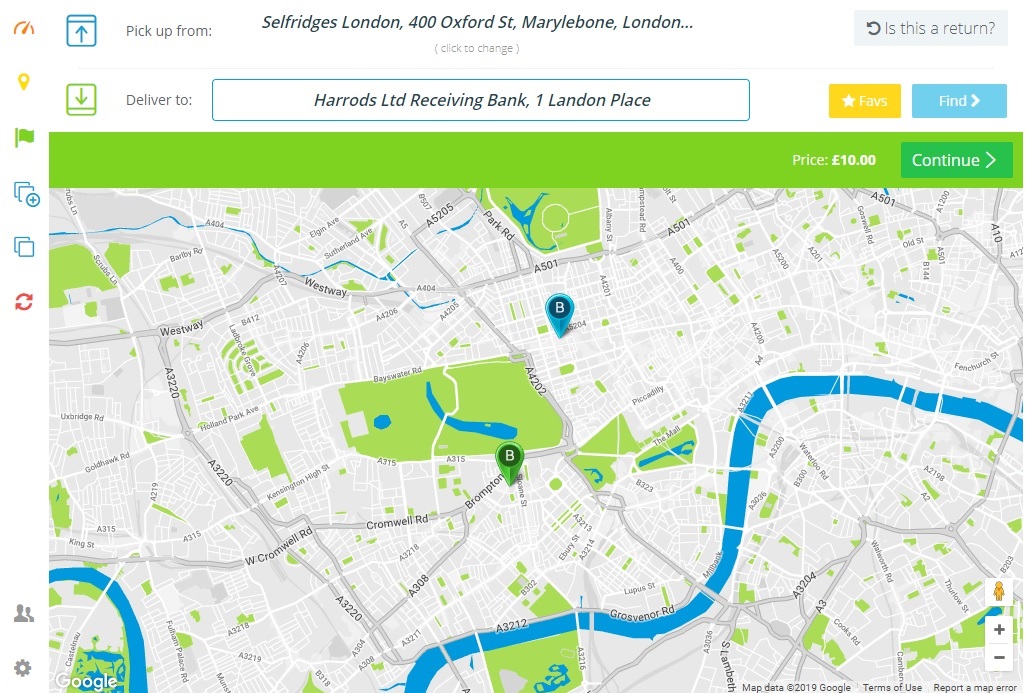This image displays a map interface, resembling Google Maps, though its exact identity is unclear. The screen is longer than the visible area, featuring a large map at the center. At the top, there is a prominent green bar with text indicating "Price: Ten Pounds," accompanied by a green "Continue" button on the upper right. In the lower left corner, a Google icon is visible. At the bottom right, text states "Map data 2019 Google. Terms of Use. Report a map error."

The map highlights two points, both marked with a circle containing the letter "B." One marker is green, situated towards the center, while the other is light blue, located to the north and slightly to the east. Above the map, text reads "Pick Up From" and "Deliver To." The "Pick Up From" section, represented by a box with a blue upward-pointing arrow, lists the address as "Selfridges London, 400 Oxford Street, Marylebone, London." The "Deliver To" section, symbolized by a green box with a downward-pointing green arrow, indicates the address "Inherits Limited, Receiving Bank, One Land And Place."

The image appears to depict a delivery application interface, illustrating the route and details of a delivery from one location in London to another.